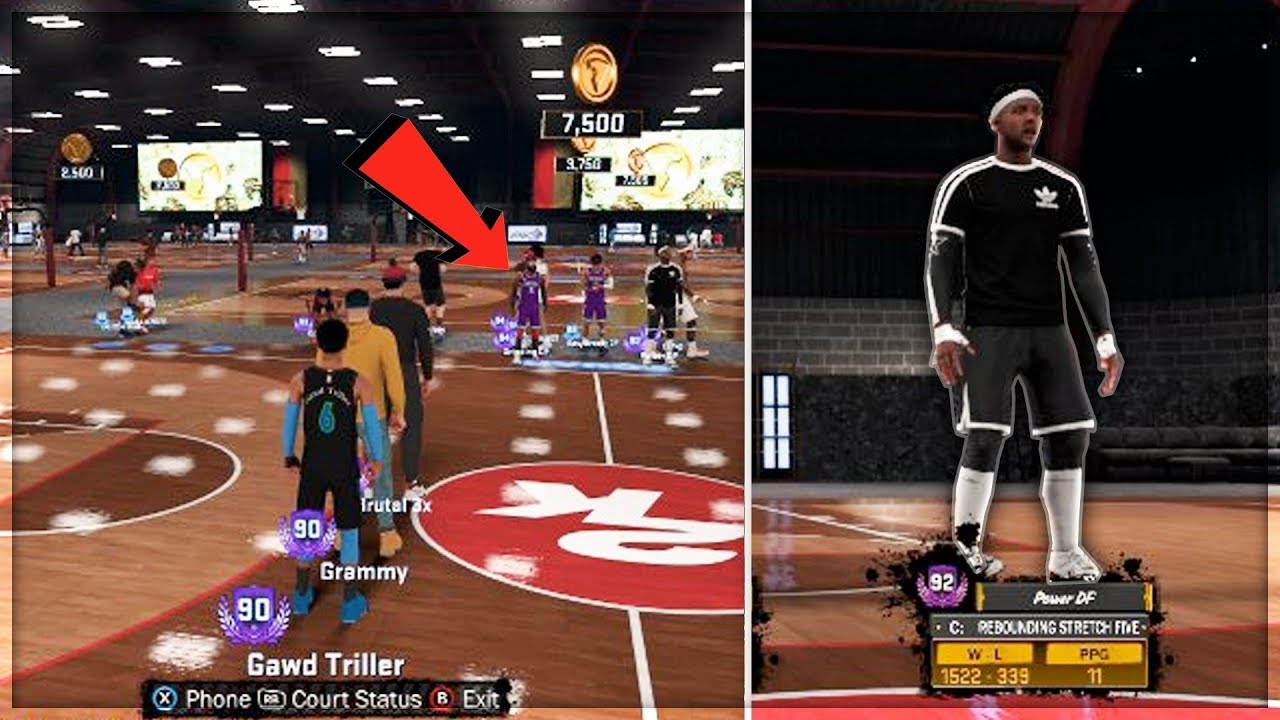The provided image consists of two distinct sections. 

**Right Side Image:**
The right section features a detailed portrait of a dark-skinned man standing in what appears to be a basketball court. He sports a black and white Adidas shirt layered over a black shirt. His attire includes black shorts with black leggings underneath, white socks, and white shoes. He also wears a white bandana on his head and has short black hair. The background reveals gray brick walls and a basketball court floor, which is a mix of light brown, dark brown, and red hues with red and white lines. There's a black and gray box at his feet displaying his stats. At the top, the text in white reads "Power GF," accompanied by a purple circle with the number "92" in white text. Below "Power GF," it likely mentions "Rebounding Strength" and there are two other yellow boxes.

**Left Side Image:**
The left section showcases a broader view of the basketball court, populated with several individuals seemingly organized in a line. The central figure dons a black tank top with blue sleeves, blue leggings, and blue shoes. Behind him, a man in a yellow shirt with blue pants stands, and in front of them, a person in a black outfit paired with a red cap is visible. The background also features various basketball players, notably a player in a purple outfit on the right, indicated by a large red arrow pointing towards him. The court’s floor shares the same dark brown and light brown pattern, interspersed with white and red lines. Additionally, there is a red circle marked on the ground in the bottom-right corner.